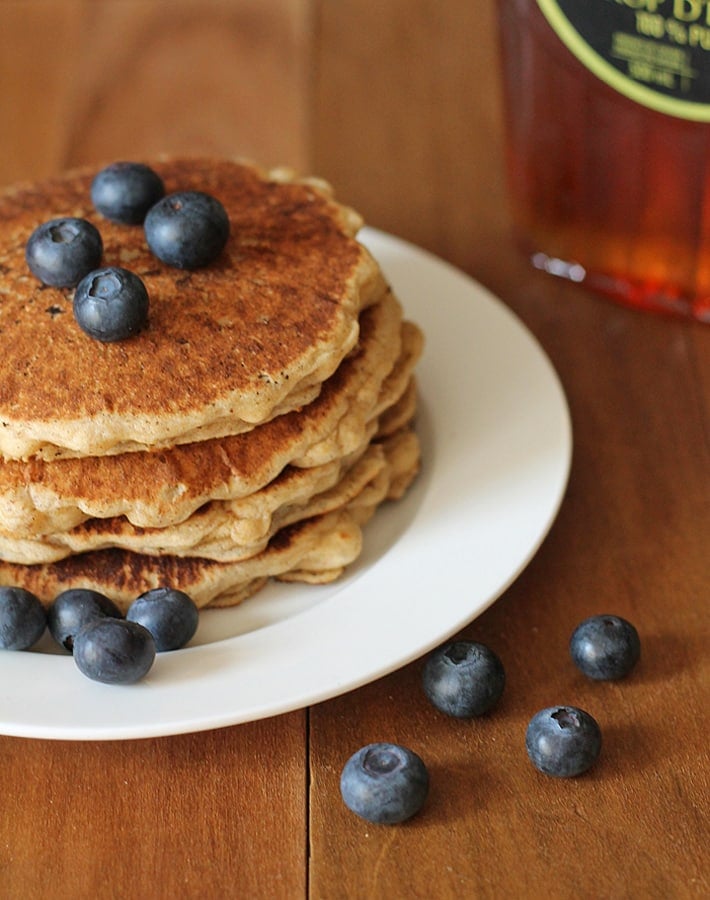A close-up photograph showcases a stack of four whole grain pancakes, marked by their golden-brown tops and lighter tan, rustic edges. Flecks of black pepper the slightly uneven, round pancakes, suggesting a whole grain texture. The stack sits centered on a white plate that rests on a wooden table. Placed delicately atop the pancakes are four fresh blueberries, and another four blueberries adorn the plate in front. Additionally, four fallen blueberries lie just off the plate on the table, adding to the charm of the scene. A partially visible bottle of syrup peeks from the top right corner, featuring a label with a gold border and a classic amber hue, albeit blurred and slightly obscured. This detailed setting captures a rustic breakfast moment, blending textures and colors seamlessly.